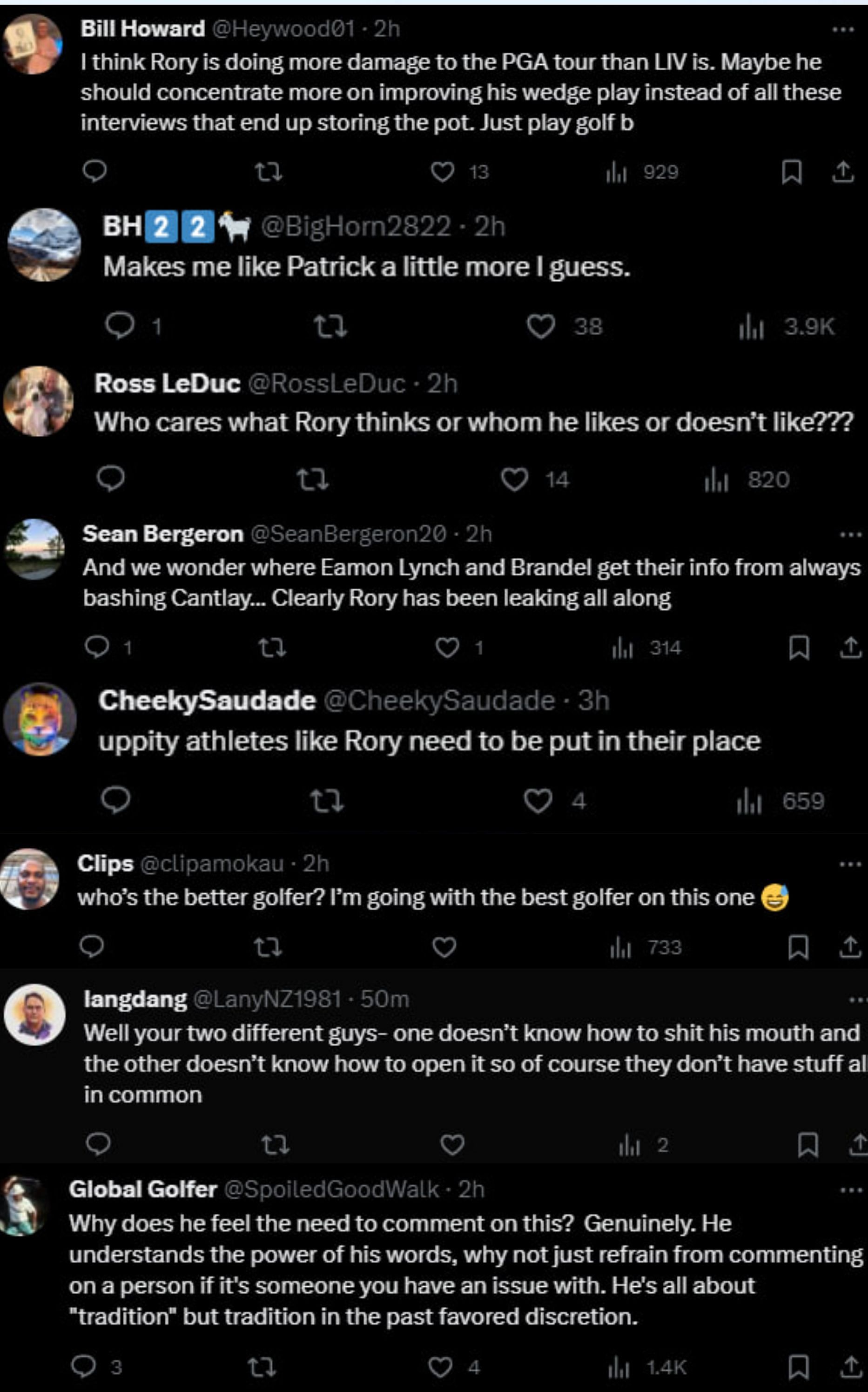The image is a mobile screenshot of a conversation thread on the social media platform formerly known as Twitter, now rebranded as X. The user is browsing in dark mode, providing a black background with white text, immediately drawing attention to a back-and-forth exchange among various people discussing professional golf, specifically the ongoing feud between PGA Tour and LIV Golf. 

The conversation kicks off with Bill Howard, who posted two hours ago, saying, "I think Rory, referring to Rory McIlroy, is doing more damage to the PGA Tour than Liv is. Maybe he should concentrate more on improving his wedge play instead of all these interviews that end up stirring the pot. Just play golf." 

The next comment reads, "Makes me like Patrick a little bit more I guess," likely referring to Patrick Reed. Ross LeDuc chimes in with, "Who cares what Rory thinks or whom he likes or doesn't like."

Sean Bergeron adds a layer of intrigue by saying, "And we wonder where Eamon Lynch and Brandle get their info from anyways bashing Cantlie. Clearly Rory has been leaking all along." 

Cheeky Sudeid comments, "Uppity athletes like Rory need to be put in their place," adding a controversial perspective. Clips then asks, "Who's the better golfer? I'm going with the best golfer on this one," sparking further debate. 

Additional responses in the thread continue this passionate discussion, showcasing the divided opinions among fans regarding the influence and actions of elite golfers in the PGA-LIV rivalry.